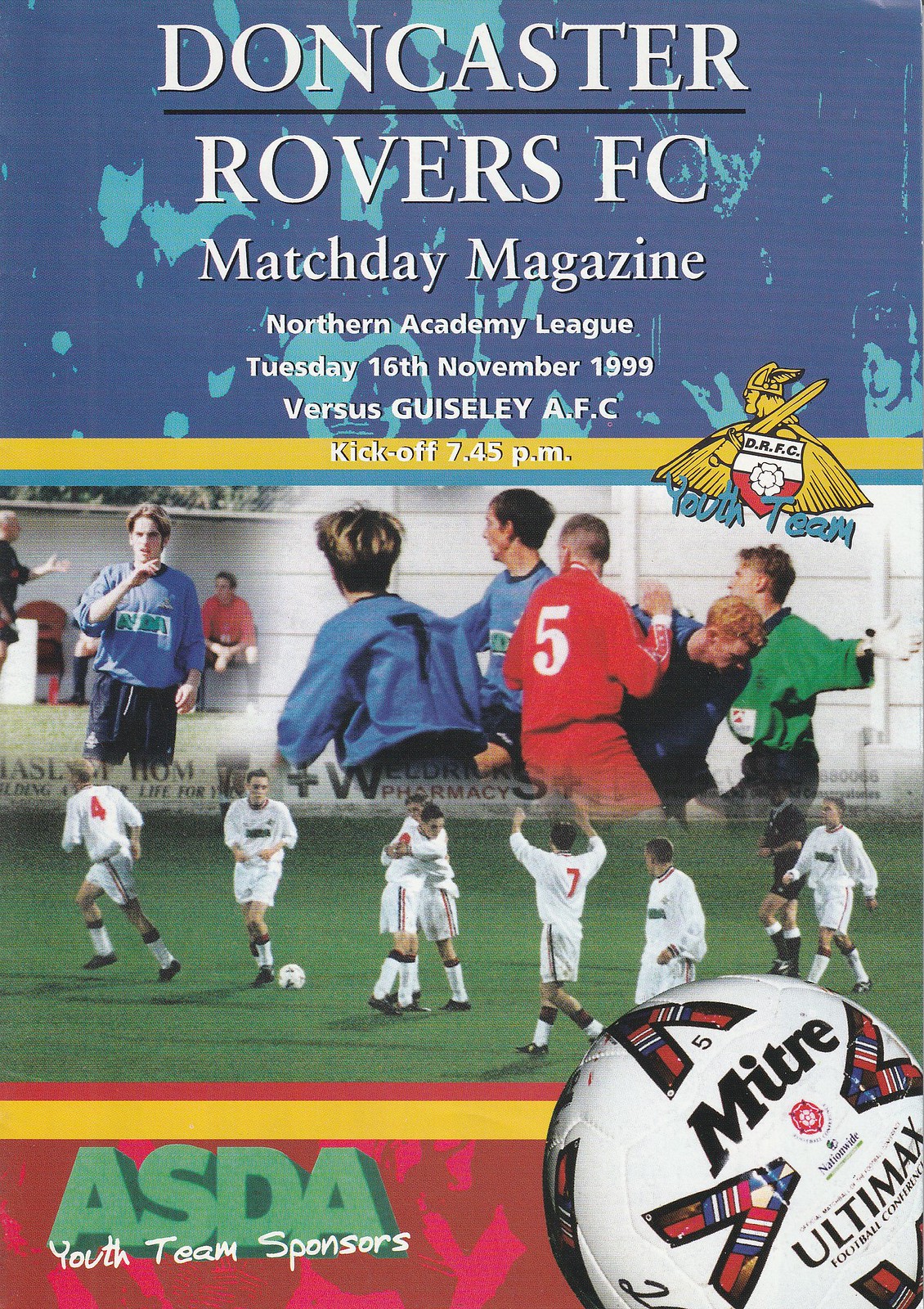This is the front page of a "Match Day Magazine" for the Doncaster Rovers FC, specifically for a match in the Northern Academy League. The event occurred on Tuesday, November 16th, 1999, with a kickoff time of 7:45 p.m. against Guiseley AFC. The top of the page prominently features the title and essential event details in white lettering on a blue background, with "Doncaster Rovers FC" and "Match Day Magazine" prominently displayed. Below this is a striking yellow stripe that leads into the main section, which consists of two separate rectangular photographs of soccer players in white and red uniforms during a match on a green field. 

At the bottom of the page, in green text set against a red background with another yellow stripe, it says "ASDA Youth Team Sponsors." The bottom right corner features a Mitre Ultimax soccer ball with the number five on it. Additionally, part of the layout includes a Viking logo, adorned with a helmet and cape, associated with the youth team in blue. The design incorporates a mix of colors including red, yellow, blue, turquoise, green, brown, gray, black, and white, presenting a vivid and dynamic visual style fitting for a sporting event flyer.